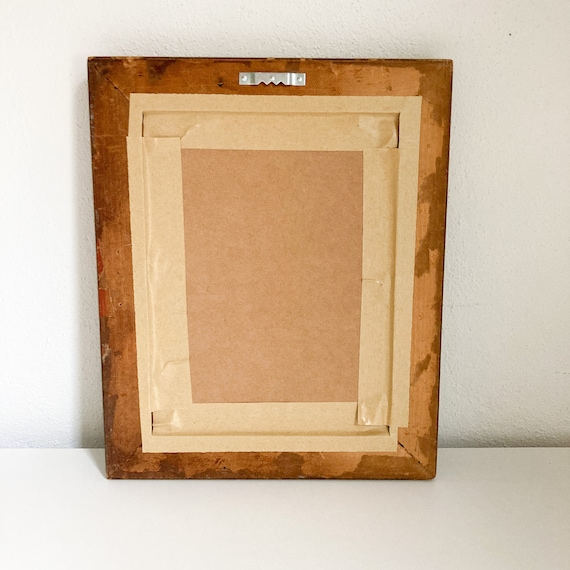This colored photograph, which is vertically rectangular with no border, was taken indoors and appears to be meticulously staged. The background comprises a gradient of gray, with the left side being lighter due to a strong light source that almost washes it out, and the right side being significantly darker. About 20% up from the bottom, a vertical line bisects the image, drawing attention to the main focus: the back of a wooden picture frame.

The wooden frame, prominently displayed in the center, reveals various intricate details. The frame itself is made of dark wood, encasing a lighter wood surrounding a central area that seems to be made of cardboard. The cardboard back is secured in place with staples, and there are noticeable splotches of glue scattered across it, suggesting a lack of attention to the hidden side of the frame. Masking tape is also visible, haphazardly placed around the cardboard base to hold it together.

At the top of the frame, there's a small hook designed for hanging the frame on a nail. This hook, along with the rough assembly of tape and glue, highlights the typically unseen, utilitarian side of the frame. The overall setup against this plain, somewhat gradient backdrop may suggest that the image was intended for online marketing, showcasing the back construction details of a frame that might otherwise be overlooked.